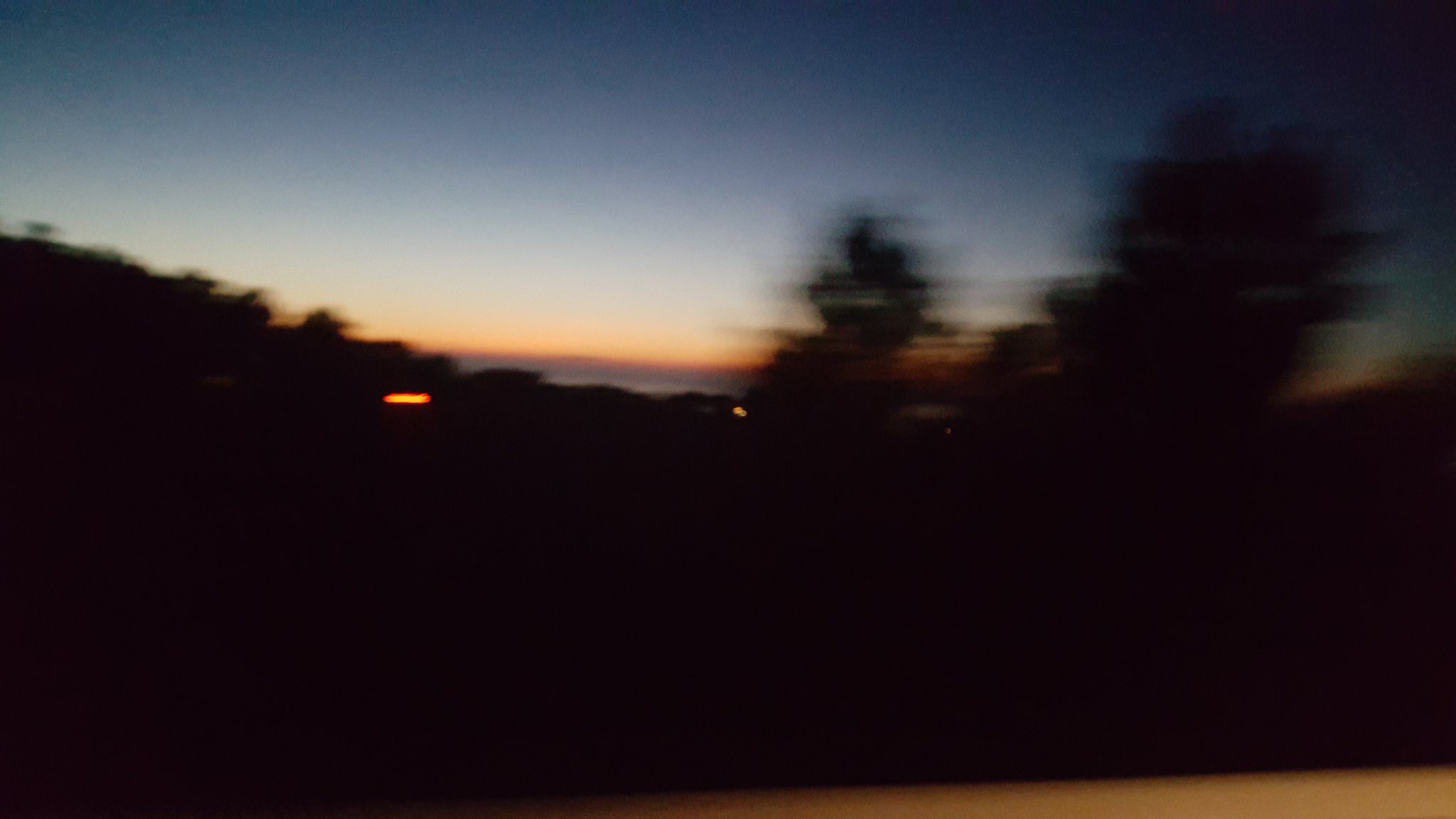The image is a blurry photograph taken at dusk, shortly after the sun has set, from what appears to be a moving vehicle. The horizon still holds traces of light, with the sky transitioning from a deep blue at the top to an orange and golden hue near the center, indicating the recently set sun. The scene features dark silhouettes of trees scattered across the middle ground and a faintly visible road at the bottom edge. To the left of center, there's a small, reflective orange bar of light on the landscape, while another dot of yellow light can be seen in the distant center. The overall setting is simple but captures the essence of an outdoor, naturally lit post-sunset environment, with minimal visible details beyond the colors of the sky and the dark shapes of trees.